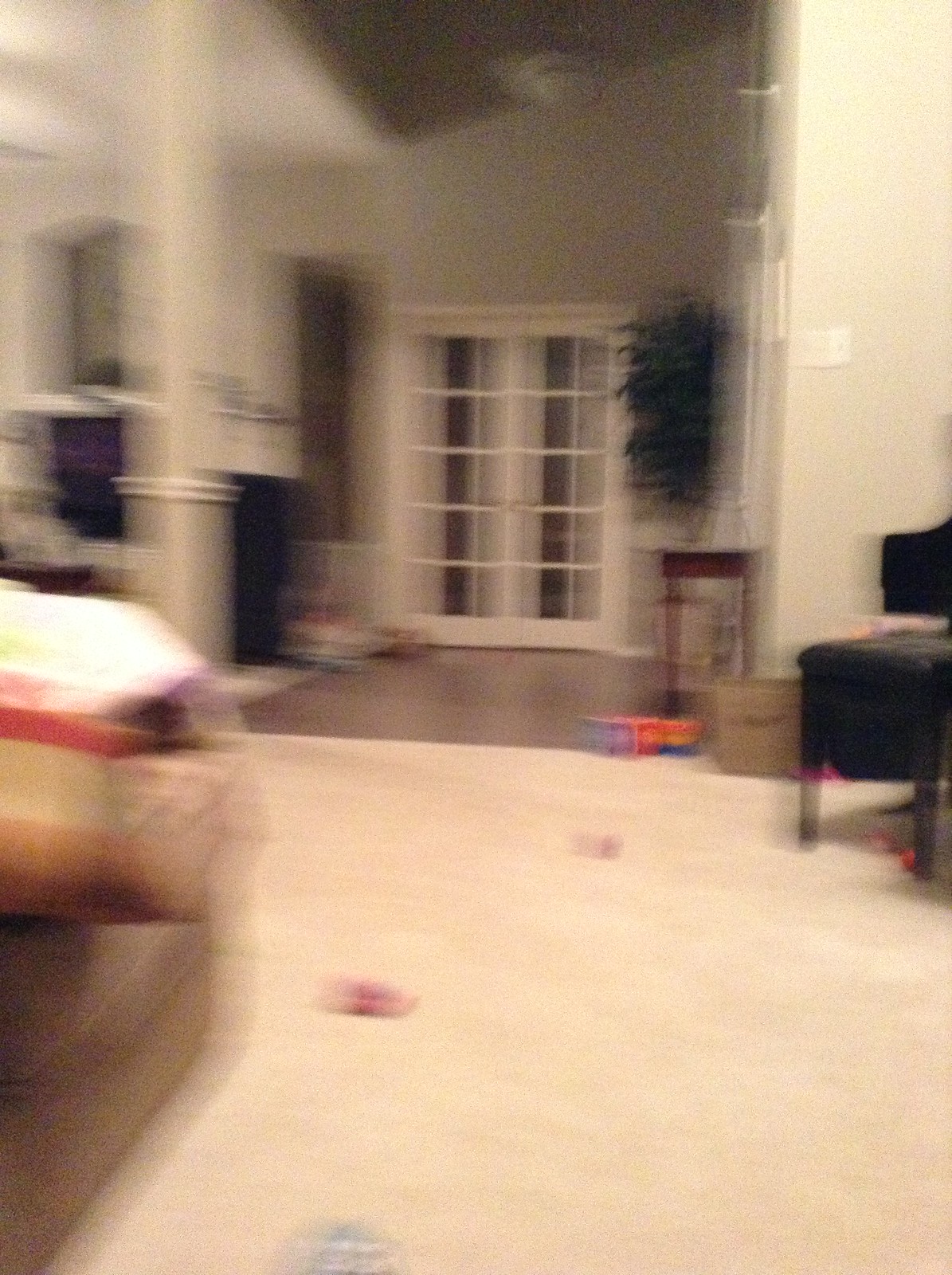The image depicts a highly blurred interior room where details are challenging to discern; however, some elements are identifiable. At the center, there are beige walls and a set of French doors adorned with curtains, suggesting an entrance to an outside area bathed in light tan hues. Adjacent to these doors on the right is a tree, possibly a houseplant, accompanied by a small table. In the right part of the image, a dark-colored chair is visible. To the left, partially in the foreground, there appears to be the side of another chair or perhaps a piece of furniture like a fireplace. This fireplace, positioned just left of the French doors, features a black section near a column. Various toys or items are scattered on the floor, adding to the room's lived-in ambiance.